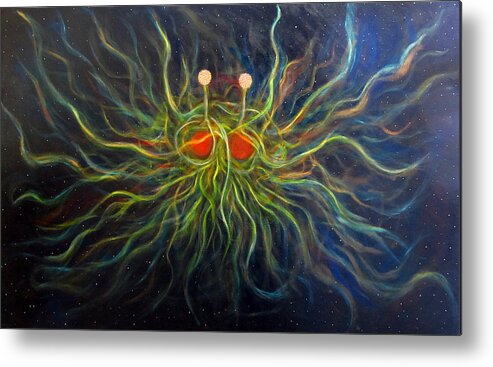This image depicts a small, horizontally aligned rectangular artistic print, slightly angled to reveal a thin depth on the right side, possibly implicating a canvas. Dominating the scene is a bizarre, Cousin-It-like creature with a central position, featuring large red or orange circular shapes that appear to be eyes. However, there is a debate that these could alternatively be cheeks or ears, as two smaller orange eyes reside atop slender green stems resembling antennae. The creature’s woolly, multicolored hair radiates in all directions, transitioning in hues as they spread out—green, brown, yellow, orange, and light red, with some even appearing blue towards the edges. The background creates a cosmic atmosphere, transitioning from dark blue to black with speckles of white mimicking tiny stars, while a bluish-brown tint appears on the right side and across the top of the composition.